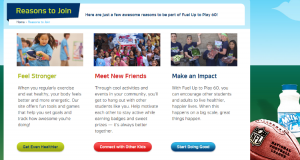This image is a small, low-resolution screenshot of a website, appearing almost as small as a postage stamp on my screen. At the top of the image, there is a navy blue rectangle located in the upper left corner containing the text "Reasons to Join" in white font. This is juxtaposed against a white rectangle, and to the right of this, there is some unreadable black text. The background of the website features a cartoon-like illustration of a blue sky. 

In the lower left corner of the image, there's a graphic that depicts green ground underneath the sky background, though it appears poorly rendered. The graphic also includes an unusual combination of an NFL football and a bottle of milk. 

Below the white rectangle, there are three distinct photos each accompanied by a short paragraph. The first photo is captioned "Feels Stronger" and depicts a little girl running. Each element of this screenshot contributes to an overall impression of a website providing some sort of promotional content or membership-related information.